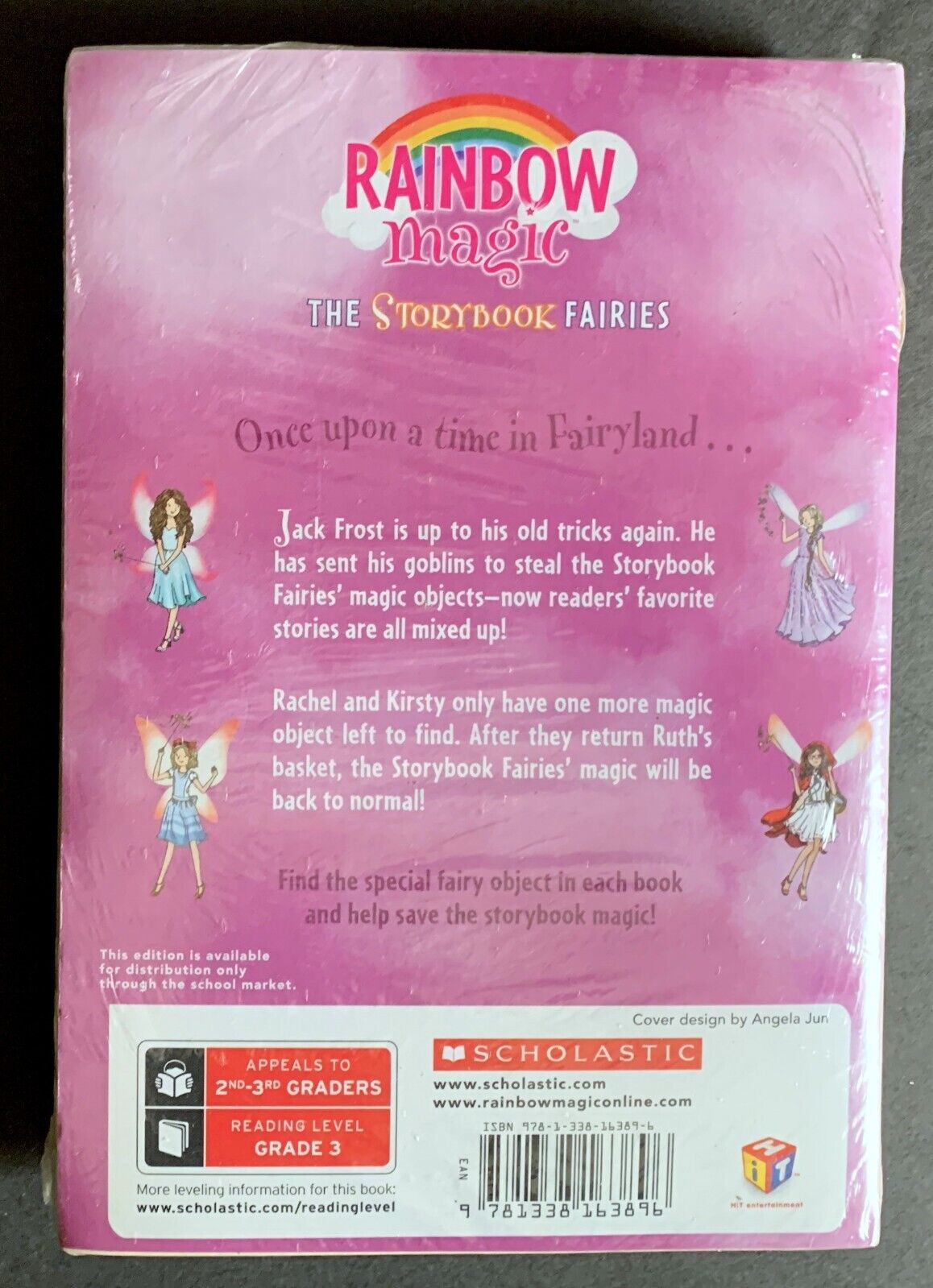The cover of the children's book, photographed in portrait orientation, features a vibrant pink background interspersed with wispy white clouds and framed by a light gray border. At the top, a vivid multicolored rainbow arches between two white clouds. Overlaying the rainbow in bold pink text is the title "Rainbow Magic," followed by "The Storybook Fairies," with "storybook" in yellow and "fairies" in white.

Positioned beneath this, a purple text reads, "Once Upon a Time in Fairyland..." Below this narrative teaser, two paragraphs of white text detail the whimsical plot: "Jack Frost is up to his old tricks again. He has sent his goblins to steal the storybook fairies' magic objects. Now, readers' favorite stories are all mixed up." The second paragraph continues, "Rachel and Christy only have one more magic object left to find after they return Ruth's basket. The storybook fairies' magic will be back to normal."

Flanking the text are four fairy illustrations—two on each side, arranged vertically. The upper-left fairy has dark hair and wings, while the lower-left fairy sports blonde hair and a blue dress. On the right, the upper fairy wears a purple dress with long braided hair, and beneath, a fairy dons a red overcoat over a white dress. Each fairy illustration is detailed, capturing the magical essence of the characters.

Towards the bottom, a white horizontal rectangle with an orange stripe reads "Scholastic" in white text next to an illustrated open book. To the left are two orange rectangles with white text: "Appeals to Second and Third Graders" and "Reading Level Grade 3." Below these details, it includes the barcode and information on the cover's designer, Angela June. The design is richly colorful and detailed, aiming to attract its young audience through the enchantment of the fairy tale motif.